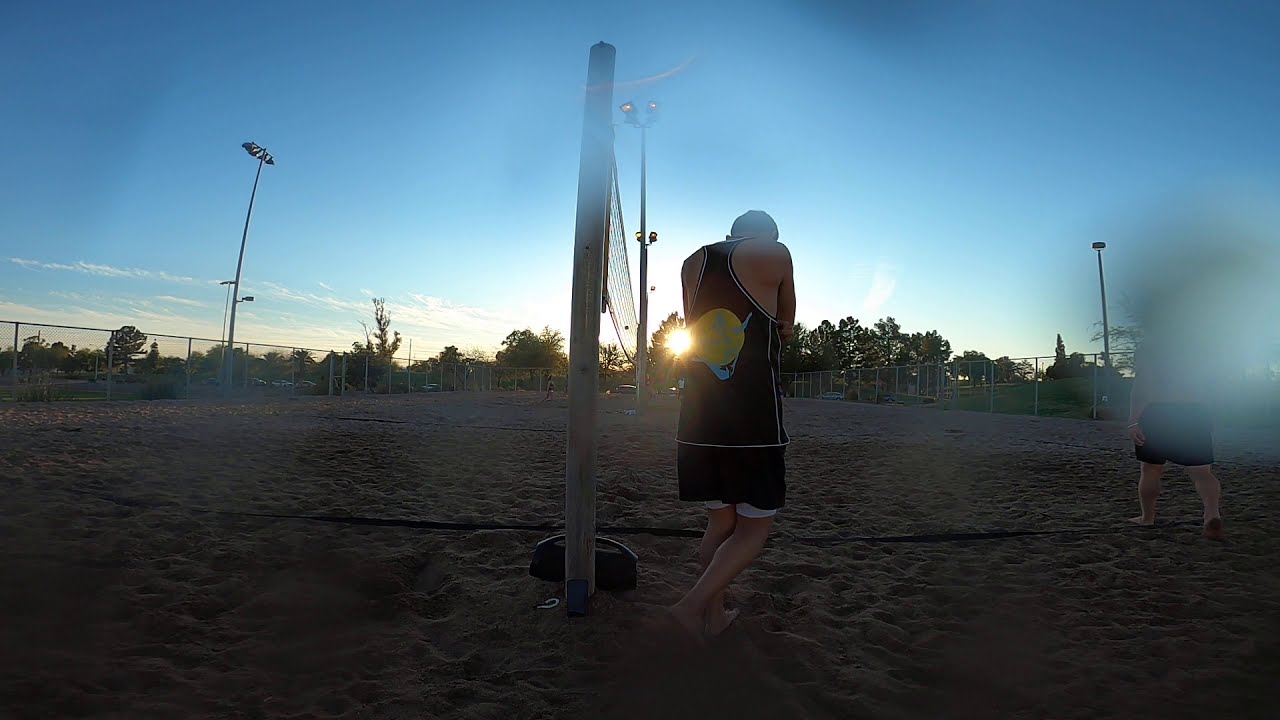The image captures a somewhat dreamy, slightly blurred scene of an evening at an outdoor sandy volleyball court. At the center of the frame, there is a volleyball net stretching out from a pole. In the foreground, the scene includes a man standing with his back to the camera, dressed in a black tank top and black shorts. He appears to be preparing to engage in the game with his arms poised for action. To the right, another man's figure is partially obscured by a possible raindrop or lens flare; he is seen wearing blue shorts. Above the sandy court, three tall light posts loom, prepared to light up the area as dusk approaches. The sky is a soft blue with a few sparse clouds, and the sun is low on the horizon, suggesting the time is either sunrise or sunset. The backdrop features tree lines that frame the volleyball court, adding a serene border to the energetic scene playing out in the foreground.